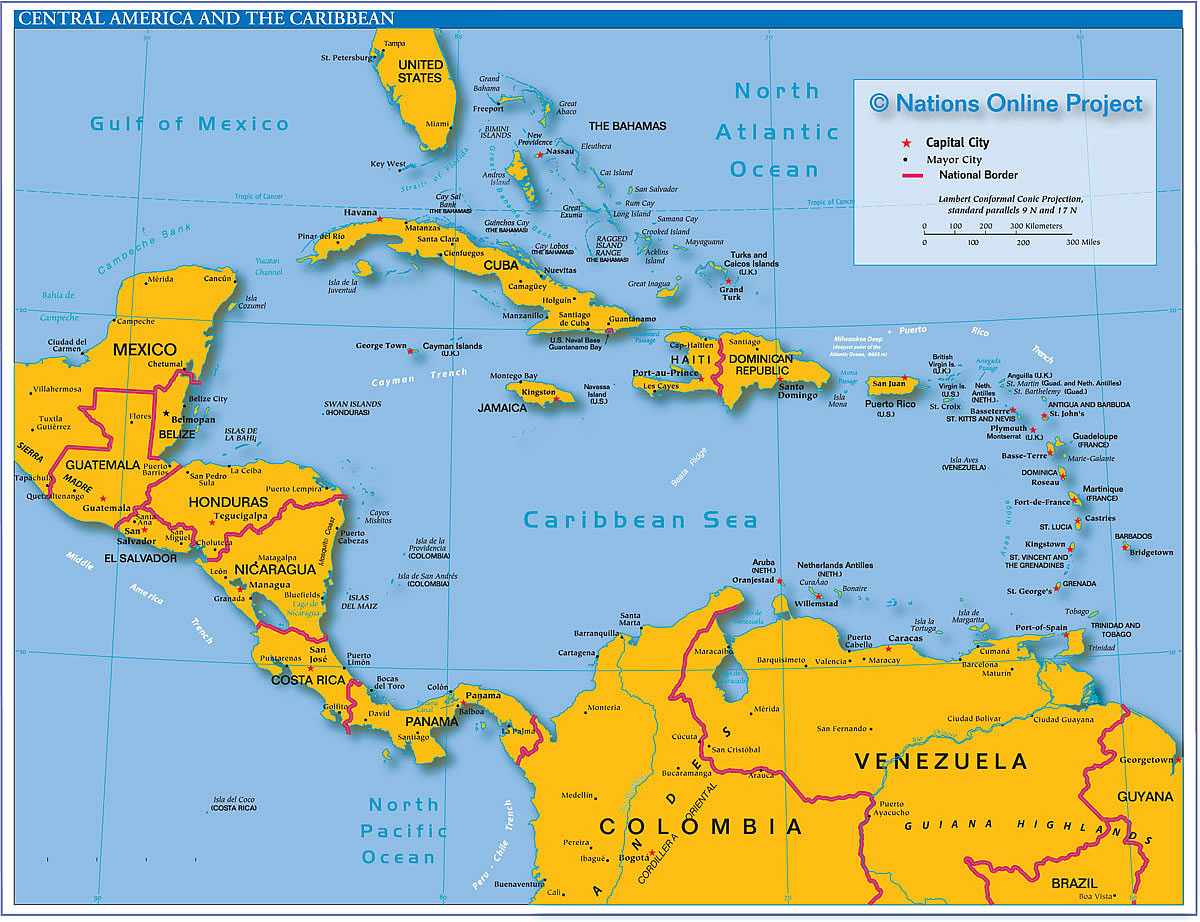This image is a detailed map titled "Central America and the Caribbean," featuring a dark blue banner with white letters. The map, sourced from the Nations Online Project, is rich with geographical detail, including the southern tip of Florida at the top, bordered by the Gulf of Mexico, the North Atlantic Ocean, the Caribbean Sea, and the North Pacific Ocean. The map highlights parts of Mexico on the left and extends to include countries in Central America such as Guatemala, Honduras, Nicaragua, Costa Rica, and Panama. The bottom right features part of South America with Colombia, Venezuela, and Guyana. Yellow-colored land masses are contrasted against blue oceans, with red lines delineating country borders. Noteworthy islands such as Cuba, Jamaica, Haiti, and the Dominican Republic are centrally located. A white legend box on the right-hand side provides information on distance, borders, and capital cities, and notes the map's copyright to the Nations Online Project.